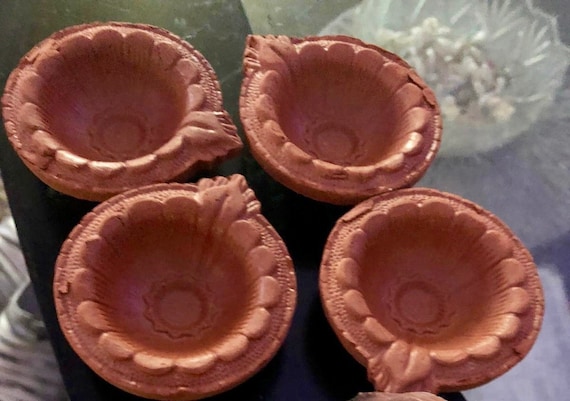The photograph showcases four identical light reddish-brown cupcake holders, each adorned with a floral print around the rim. These holders are made of plastic and are arranged in a neat two-by-two grid on a black kitchen countertop. The image, taken from a top-down perspective, also reveals a glass bowl in the blurry background. The floral designs on the rims give the holders a delicate, almost pottery-like appearance, with the center of the flower motif located at the bottom of each holder. The photograph has a slightly grainy quality, subtly blending in various shades like black, white, and gray in the background.